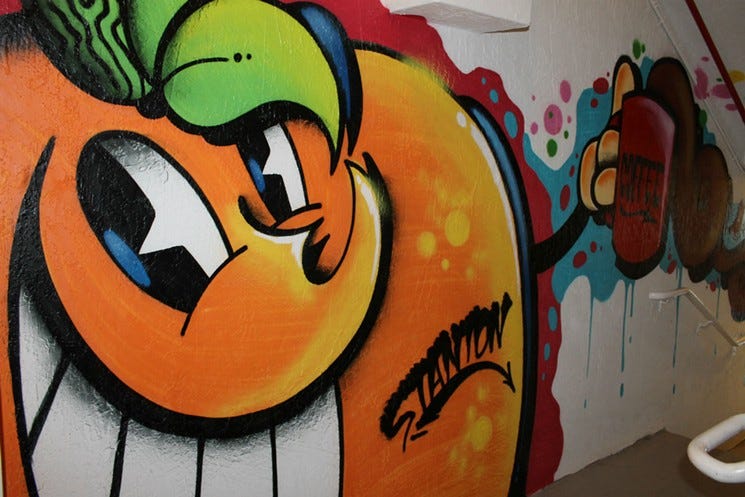The image is a horizontal, rectangular piece of art that appears to be a graffiti-style mural painted on an interior wall, possibly depicting a staircase in the upper right corner, although even the staircase might be part of the artwork itself. The focal point is a giant, round, orange cartoon character that occupies about 75% of the image. This character has a pair of upward-pointing blue eyes and a beak-like feature adorned with a set of large white teeth, though the bottom of the mouth is cut off. Atop the character's head are green leaves with blue accents. The character has a small black arm extended to the side, holding a red mug labeled "coffee" in black lettering, suggesting it's a coffee mug. Surrounding the character and in some of the image's negative space are various details like black lines, white and red dots or circles, and other color accents that fade into darker shades. Distinctive elements on the character include white oval-shaped patches, and there's a signature in black paint that reads "Stanton," likely the artist's name.